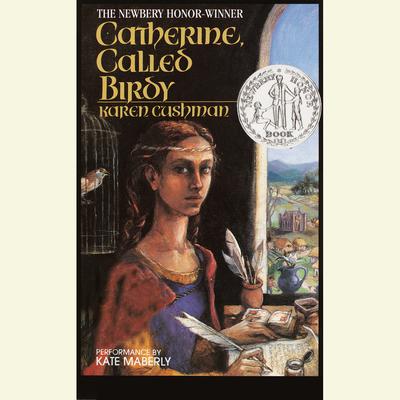This is likely the cover of a book, identified at the top as a Newbery Honor Winner. The title, "Catherine, Called Birdie," is written in yellow letters by Karen Cashman, the author's name appearing below. To the right, a thin line with a circle beside it indicates the Newbery Honor Book emblem, displaying two human figures holding hands. In the bottom left corner, in white capital letters, it notes a performance by Kate Maberly, suggesting this could be an audiobook. 

The central illustration shows a woman dressed in a blue dress with a red cape over her shoulders, seated at a table with a quill in her right hand, writing on a scroll. Nearby, there's an ink jar and a vase with additional quills. The background depicts a rural area with hills, buildings, and grass, viewed through an arched window on the right. Behind her, there's a bird in a cage. The woman, who has her hair tied in a ponytail, appears to be from a medieval period and is looking towards the viewer. The scene is rich in colors including orange, white, blue, green, yellow, gold, and silver.